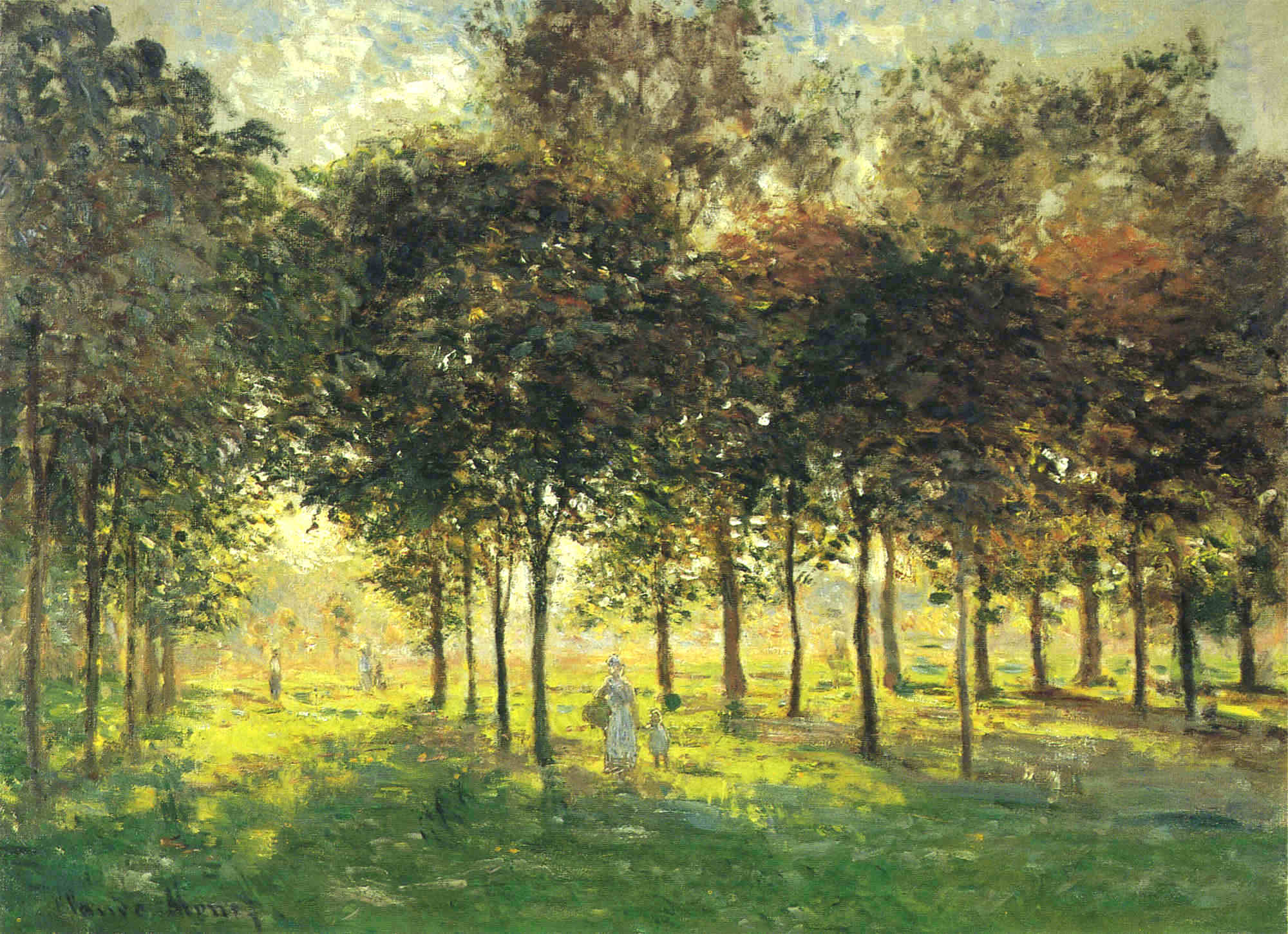The image depicts a classical oil painting of a serene park or forested area. The composition is dominated by a lush, green landscape where the ground is covered in varying shades of green grass and bushes. Tall trees with dense canopies, painted in a mixture of green and some red and brown hues, populate the scene and are lit by warm sunlight filtering through, suggesting it is daytime with a blue sky and scattered white clouds in the backdrop.

In the center, an adult woman and a child, both dressed in white clothing, are walking hand in hand. Their placement and attire draw immediate focus, while in the background, faint figures of other people can be seen, adding depth to the scene. The artist's pronounced brush strokes contribute to the texture, emphasizing the natural beauty and tranquility of this park or garden setting.